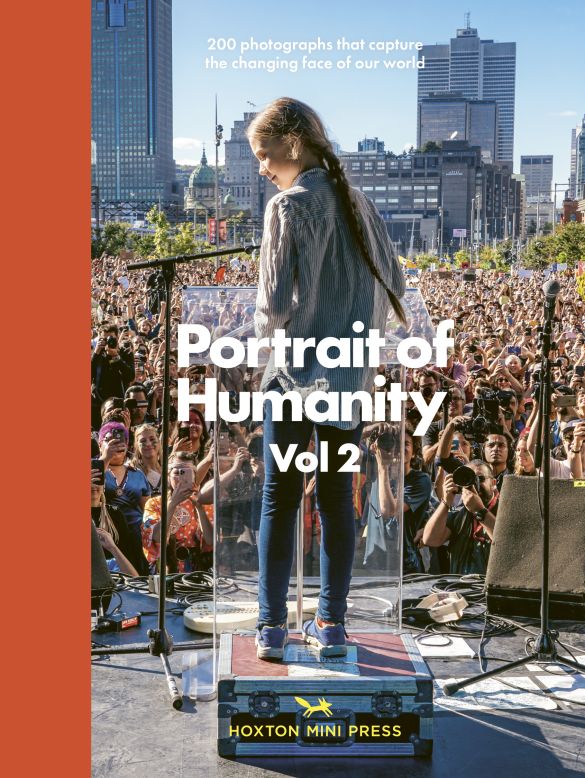The cover of "Portrait of Humanity Volume 2" by Hoxton Mini Press, featuring a small yellow fox icon, is an evocative scene capturing a young girl elevated on a podium with a microphone, speaking to a vast, enthusiastic crowd. Surrounding her are people filming with their phones and professional cameras, while many hold up signs. The background showcases a downtown area with a mix of tall skyscrapers and smaller buildings, set against a blue sky with wispy grey clouds. The crowd, filled with smiling faces and cheering kids, emphasizes the book's theme, echoed in the text at the top: "200 photographs that capture the changing face of our world."